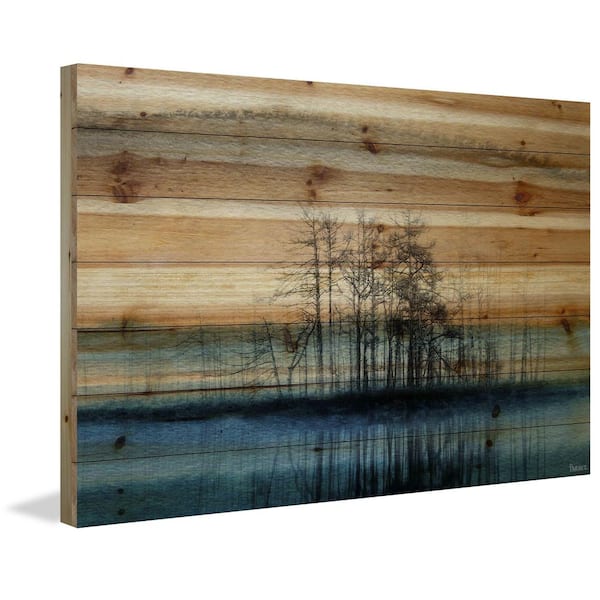Rectangular wooden canvas, depicting a gradient of colors transitioning from a bluish teal at the bottom to aquamarine, light denim blue, navy blue, and then green. The central area showcases black silhouettes of trees with intricate branches and twigs. The background behind the trees fluctuates in shades, starting with beige and light brown, repetitively layered to culminate in brown. The entire canvas is slanted, with the left side tilted towards the bottom left corner and the right side towards the upper right corner.